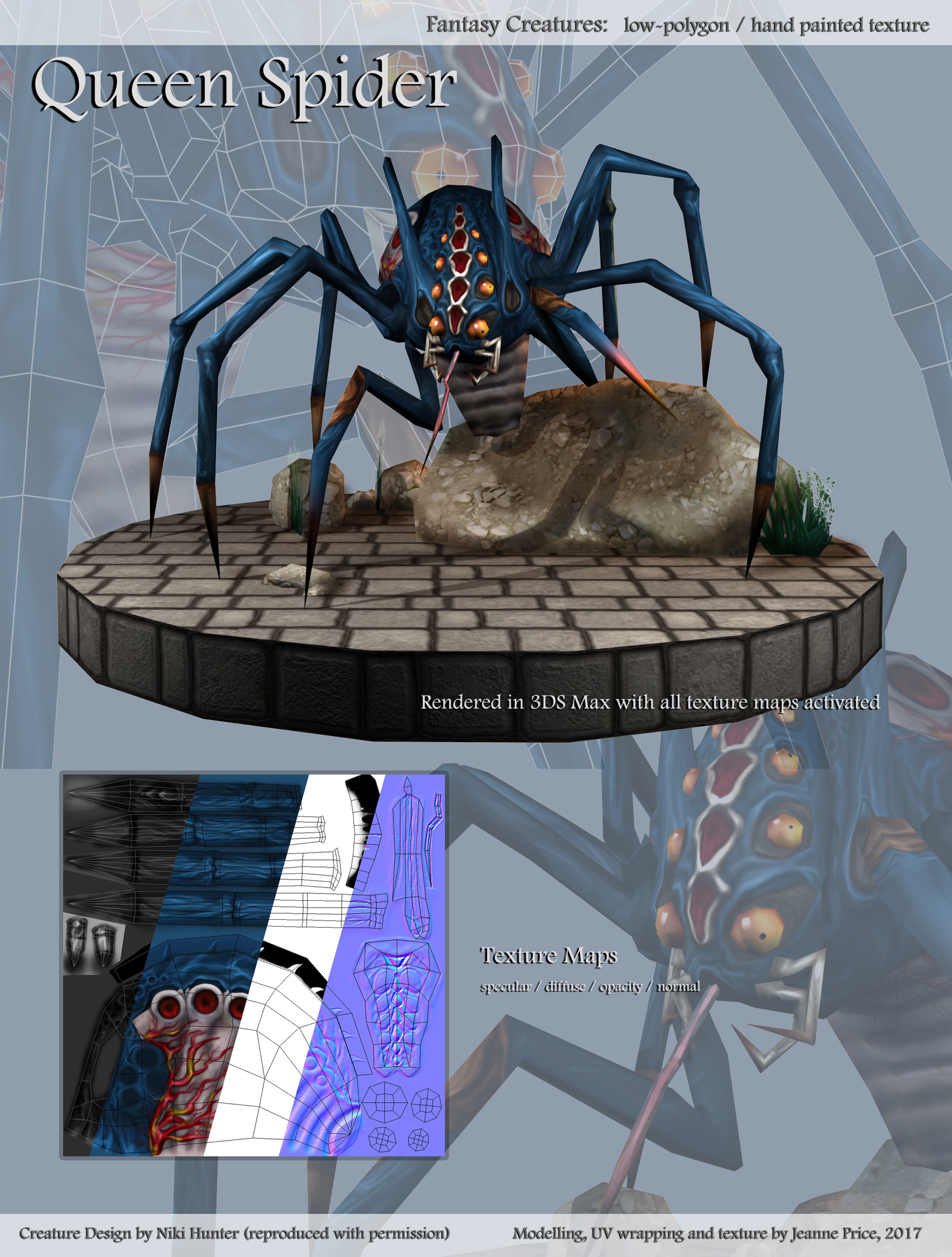The image presents a detailed computer graphics render of a fantasy creature entitled "Queen Spider," prominently labeled in the top-left corner. This color illustration appears to be part of a magazine spread focused on low-polygon, hand-painted texture models and was rendered using 3DS Max with all texture maps activated, including specular, diffuse, opacity, and normal maps. The central scene features a blue, yellow, and red spider with multiple rows of eyes, four front mandibles, and a large antenna. The spider sits atop a circular brick platform with a large rock at its center. The creature is adorned with orange dots and a middle pattern of red shapes along its back, while its legs are sharp and culminate in pointed tips. In the translucent background, lighter views of the spider provide additional perspective. Text elements and a square inset featuring an abstract design with blue, white, black, and purple colors decorate the image, contributing to its intricate and layered composition.